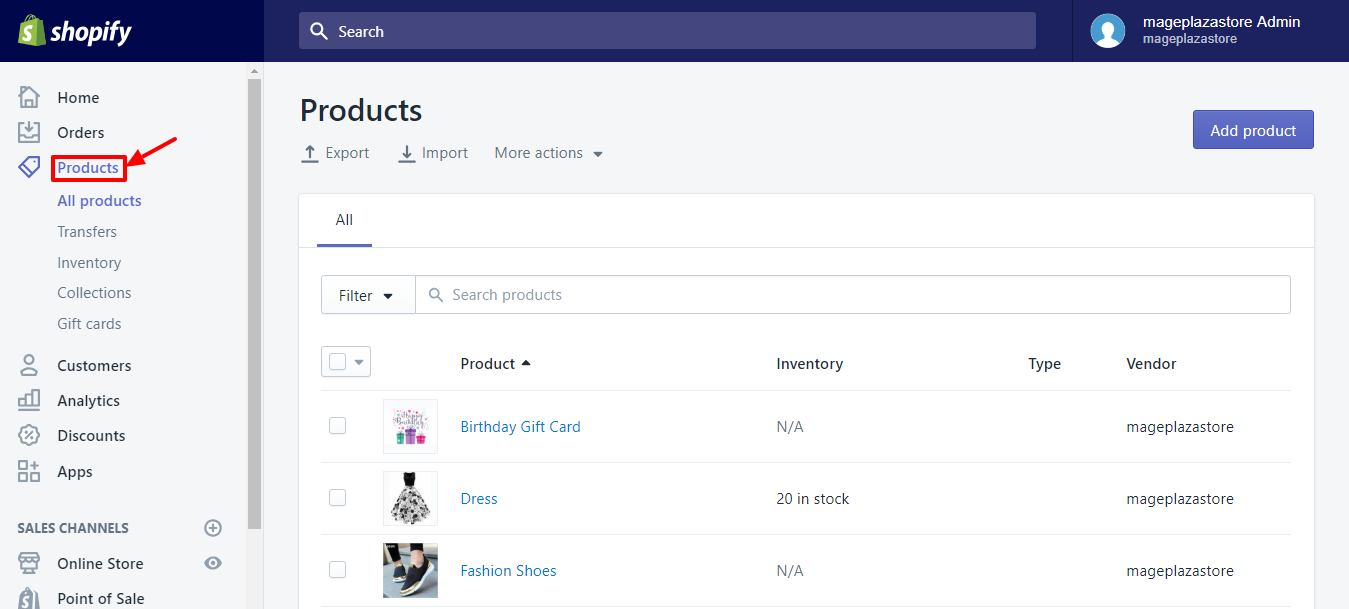Screenshot of the Shopify Admin Dashboard:
- **Top Section**: A blue rectangular box housing a large search bar labeled "Mag Plaza Store Admin."
- **Left Sidebar**: Light gray background with navigation options:
  - "Home" (black text)
  - "Orders" (black text)
  - **"Products"** (blue text, highlighted with a red box and red arrow)
  - "All Products" (blue text) under "Products"
  - Other menu items in black text:
    - Transfers
    - Inventory
    - Collections
    - Gift Cards
    - Customers
    - Analytics
    - Discounts
    - Apps
    - Sale Channels: Online and Point of Sale
- **Main Section**:
  - Actions at the top: 
    - "Choose Products"
    - "Export"
    - "Import"
    - "More Actions"
  - A blue button labeled "Add Product" to the right.
  - Search and filter options for products.
  - Listed Products:
    1. **Birthday Gift Card**:
       - Inventory status: Not Available
       - Vendor: Mag Plaza Store
    2. **Dress**: 
       - Description: Black top with a frilly hem and a multicolored skirt.
       - Inventory: 20 in stock
    3. **Fashion Shoes**:
       - Description: Resembling a pair of Keds.
       - Inventory status: Not Available
       - Vendor: Mag Plaza Store